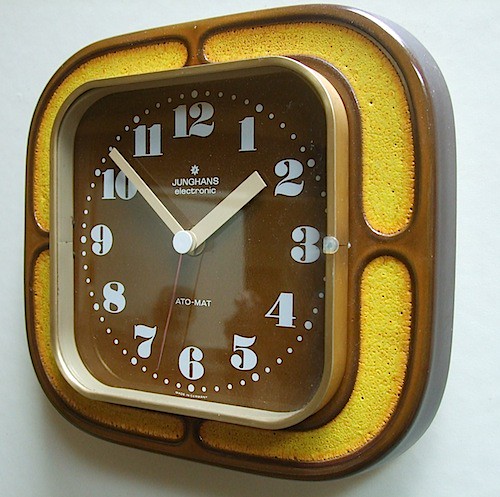The image is a detailed color photograph of a vintage wall clock. The clock has a distinctive design featuring a rounded square wooden frame with a dark walnut finish, highly varnished creating a slight reflection in the top right corner. This clock showcases a unique aesthetic with yellow foam inserts shaped like half moons running along the border. The clock face, set slightly in from the edge, mirrors the rounded square shape of the outer frame, maintaining the same excellent scale proportions.

The clock's face has large, modern-looking white numbers on a chocolate brown background, emphasizing clarity. Brand markings on the clock include "Hans Electric ATO-MIT," hinting perhaps at its Scandinavian origins, although one caption suggests the brand name might be German. The hands of the clock are distinctive: the second hand is red, standing out against the off-white beige hour and minute hands, which resemble squared-off popsicle sticks. According to the positions of the hands, the time displayed is 1:52. This clock exudes a 1970s flair with its chocolate brown and bright yellow details, making it both a functional timepiece and a decorative vintage item.